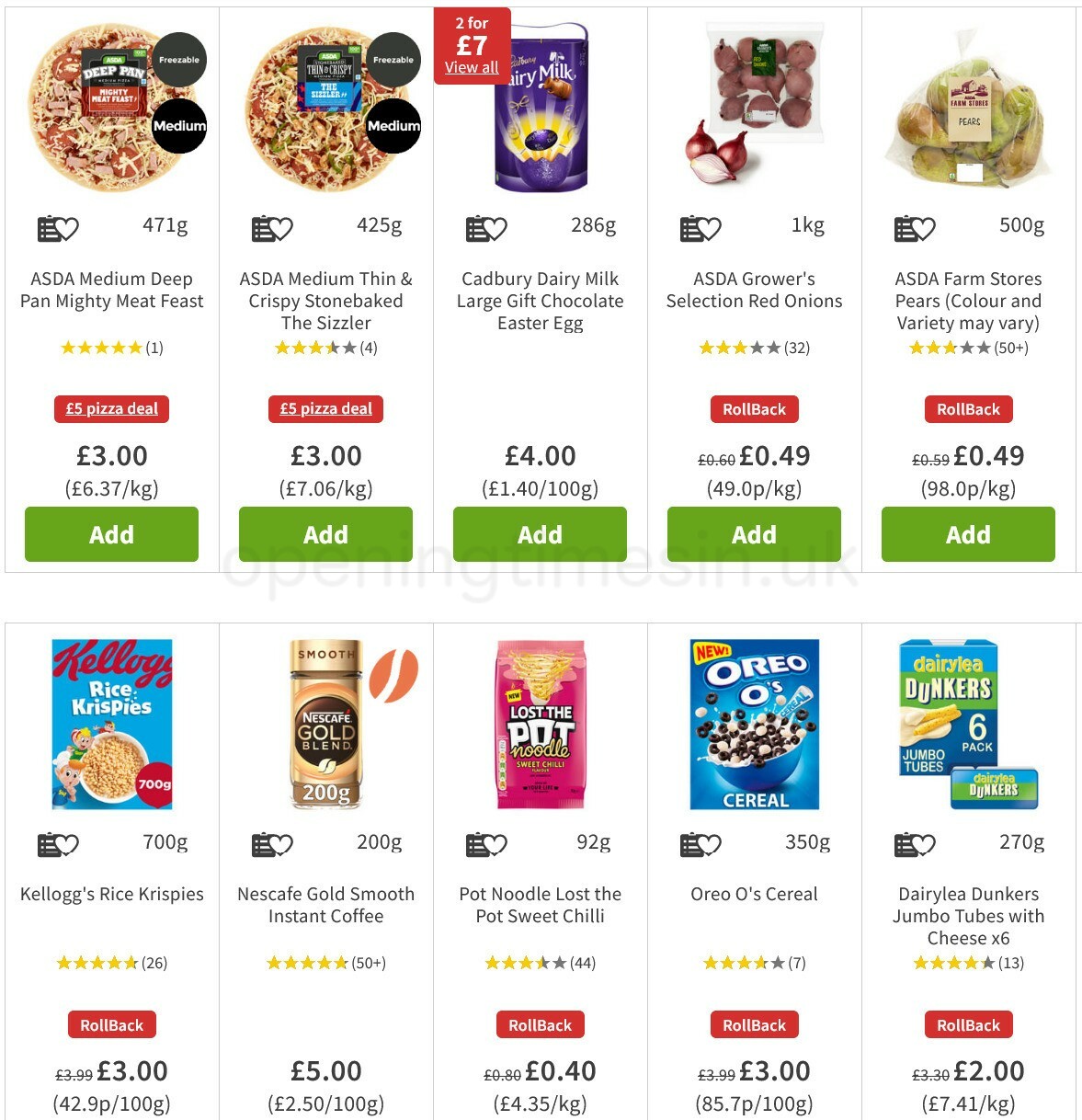A detailed description of the image:

The image displays a section of a shopping website featuring various supermarket items, all of which are food-related. The background is white, giving the page a clean and organized appearance. The items are arranged in a grid, creating a structured and rigid outline for ease of browsing. Each product is accompanied by its price, listed in British Pounds, and an "Add" button for convenient online shopping. 

Among the items showcased are several frozen pizzas, Cadbury Dairy Milk, a large gift chocolate Easter egg, red onions, pears, Rice Krispies cereal, instant coffee, instant noodles, Oreos, Dairy Milk chocolate, and a cheese snack known as Dunkers Jumbo Tubes. Some products have special indicators such as "roll back," suggesting they may be on discount or part of a promotion.